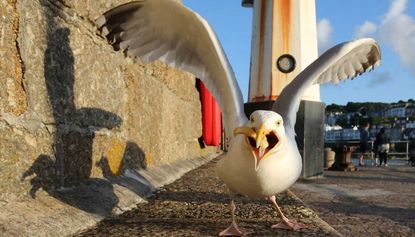In this captivating image, a predominantly white seagull with hints of gray and black on its wings is captured in mid-motion, its beak grasping a yellow worm. The gull's wings are dramatically extended upwards and outwards, giving an impression of readiness for flight. To the left, a stone wall is visible, with the seagull’s shadow cast sharply upon it. Additionally, the lower section of a lighthouse, black at the base and white above, stands behind the bird. On the right side, two individuals are seen standing in front of a metal fence, gazing out at the sea. The setting includes a concrete sidewalk beneath the seagull, contrasting with the stone road to its right. The overall composition suggests a coastal location, possibly near a bay.